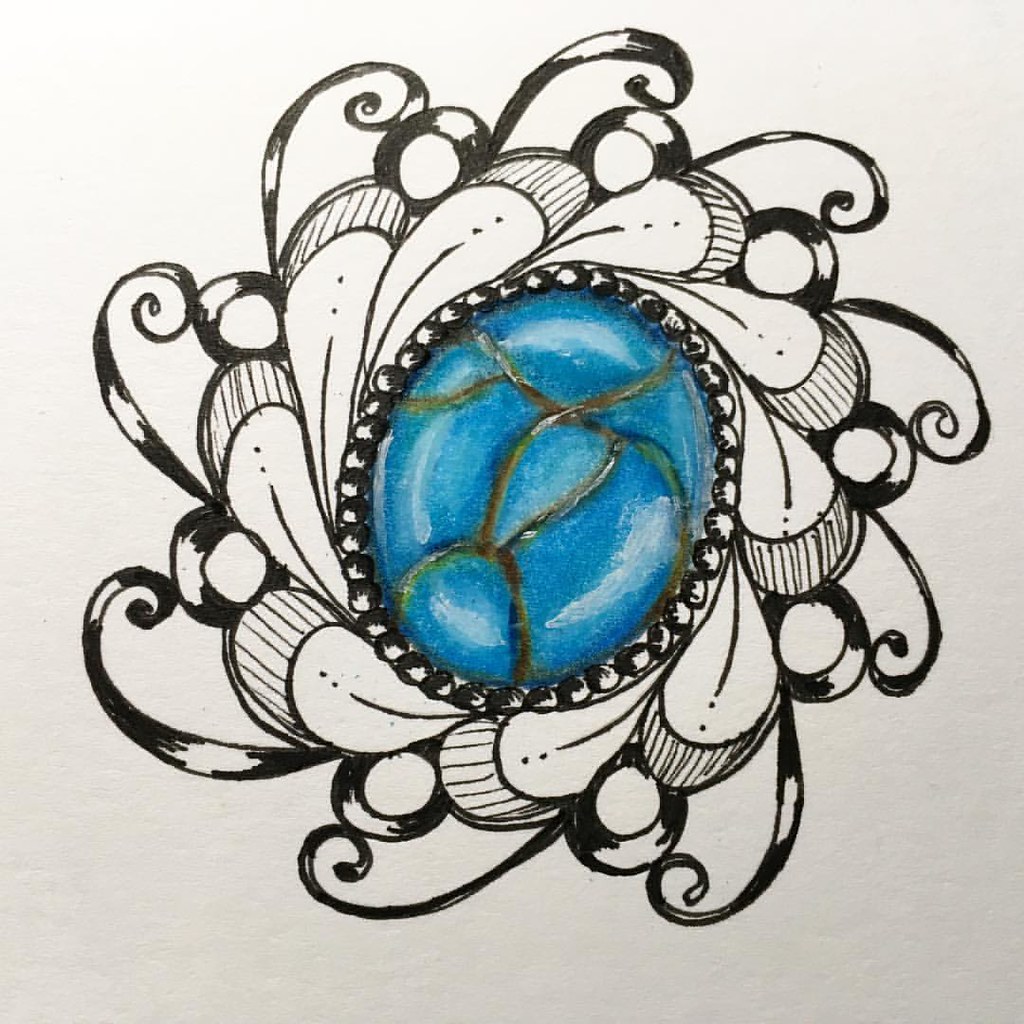This photograph captures a highly detailed and intricate drawing on what appears to be a white sheet of either sketchbook paper or printer paper. The artwork is meticulously crafted using black ink, portraying a stylized flower with petals that elegantly flow into one another, creating a harmonious circular pattern. Extending from the petals are delicate vines or subtly curved lines, adding to the organic and dynamic feel of the piece.

At the heart of this floral design lies a large, vividly colored gem, rendered in shades of blue or aqua. This gem, with its striking color, is distinguished by gold facets that add a touch of brilliance and sophistication. Surrounding the central gem are smaller, shaded circles, delicately illustrated to resemble additional gemstones or stones, enhancing the ornamental quality of the drawing.

The monochromatic petals, in black and white, contrast beautifully with the vibrant centerpiece, creating a visually captivating and balanced composition. The intricate details and careful shading suggest a high level of skill and attention to detail, making this drawing a remarkable piece of art.